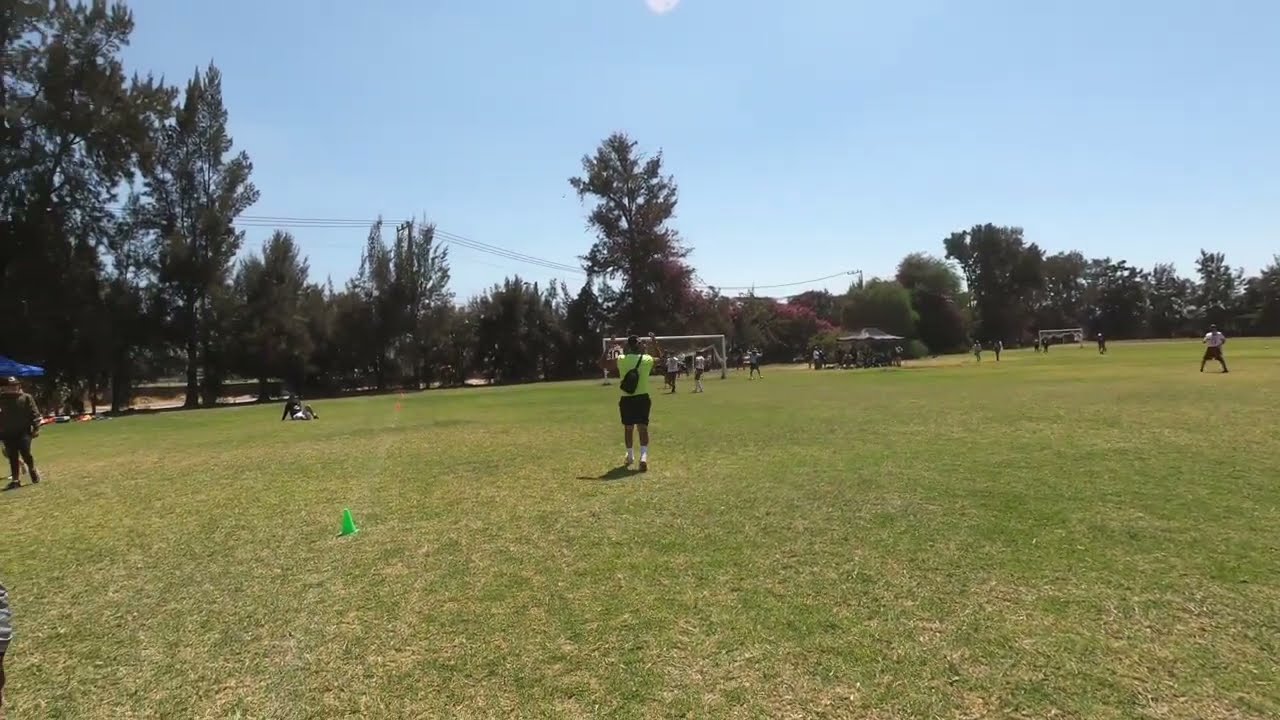In this daylight outdoor photograph, a person in a lime green shirt, black shorts, white socks, and a black side bag slung over their shoulder stands with their back to the viewer on a large, grassy soccer field. The individual appears to be either coordinating or coaching a group of predominantly teenage players who are gathered near a soccer goal positioned in the middle of the image. The sprawling field, characterized by short, mowed grass, is dotted with various people engaged in a soccer game, most with their backs turned. 

To the bottom left of the photograph, a small green cone is placed on the grass, likely marking the playing area. In the background are trees lush with green leaves, interspersed with a few red ones, lining the edge of the field. The far end also features a white cabin or bathroom to the right, power lines cutting across the scene, and another soccer field. Additionally, beneath a black tent and a blue umbrella, more observers and players can be seen. The bright blue sky with barely any clouds adds a serene backdrop to this lively park or soccer field scene.